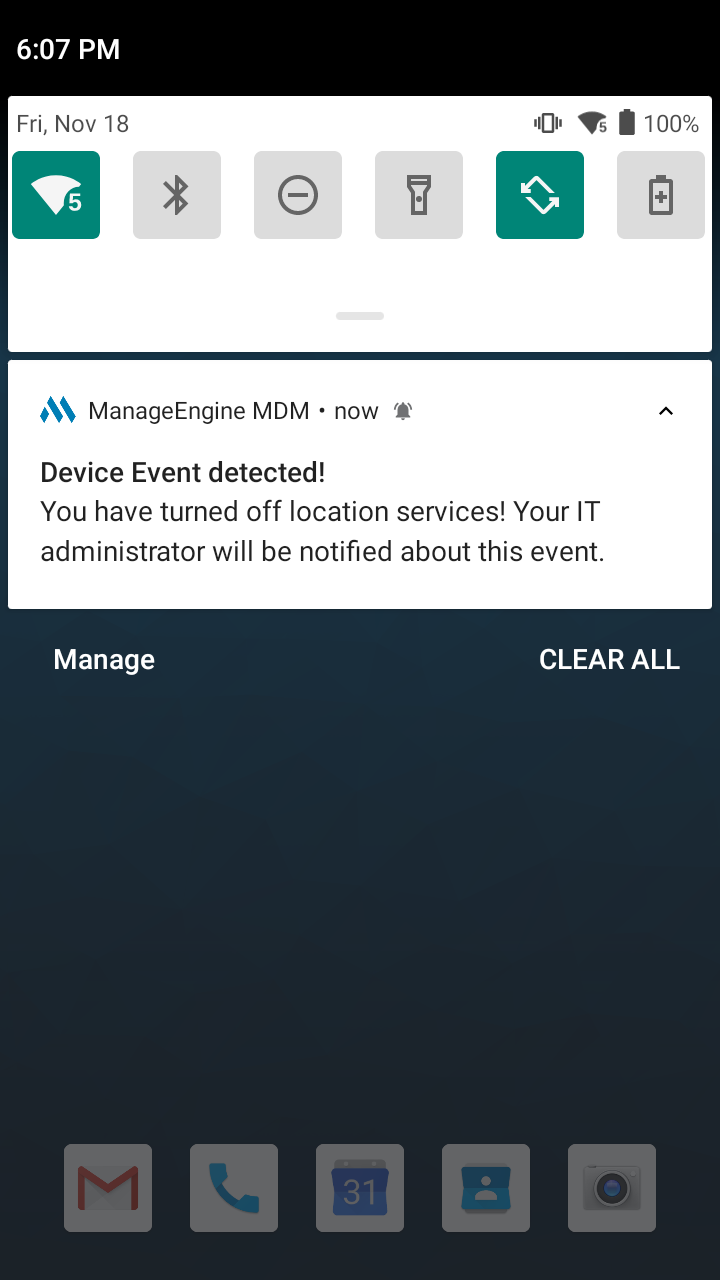A detailed screenshot captured from a cell phone at 6:07 PM on Friday, November 18, displaying a comprehensive array of system icons and a notification message from a mobile device management application. The top of the screen features standard icons indicating the status of Wi-Fi, Bluetooth, flashlight, and a full battery at 100%. The phone is set to vibrate mode.

Below the status icons, a pop-up notification from "ManageEngine MDM Now" alerts the user that a device event has been detected due to the deactivation of location services, with a warning that the IT administrator will be notified of this change. The pop-up includes options to either manage the settings or clear all notifications.

The bottom portion of the screen showcases five primary navigation icons for Gmail, Phone, Calendar, Contacts, and Camera applications. The screenshot is vertically oriented, lacking any photographic content, individuals, animals, plants, buildings, vehicles, or any other physical objects, making it a purely informational capture of the device's current status and notifications.